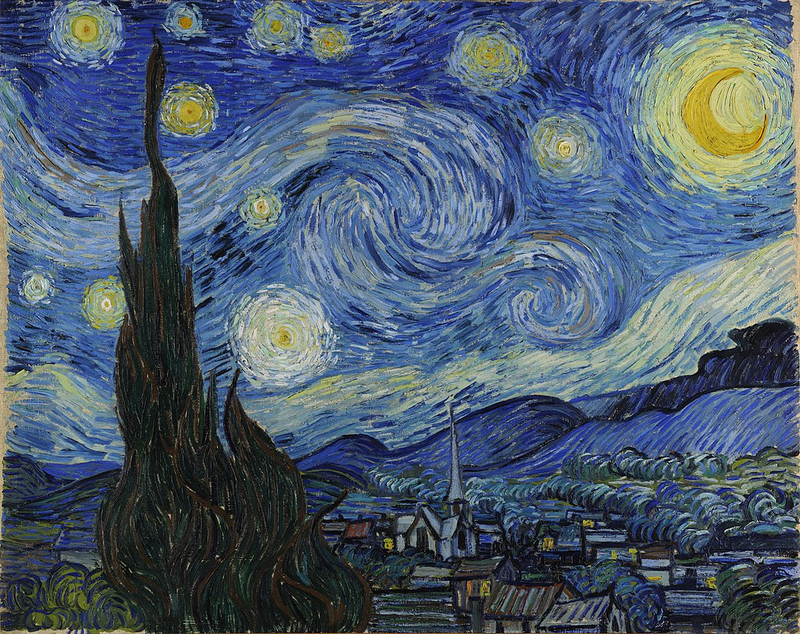This image depicts Vincent van Gogh's iconic painting, "The Starry Night," renowned for its swirling night sky and expressive color palette. Dominated by deep blues, vibrant yellows, and touches of gold, the sky is filled with dynamic, swirling clouds and radiant stars, each encircled by a shimmering halo. The large yellow orb on the right is the moon, casting its glow over the landscape. Below the celestial display lies a quaint town, with detailed depictions of small houses and prominent structures, including a church with a tall spire reaching upwards. The dark shape of a cypress tree or tower stands in the foreground, stretching towards the starry sky. The rolling hills in the background appear almost wave-like, contributing to the painting's overall dreamy and abstract aesthetic. The entire composition, possibly rendered in oil color, exudes a sense of whimsical abstraction, making it one of the most celebrated works of art.